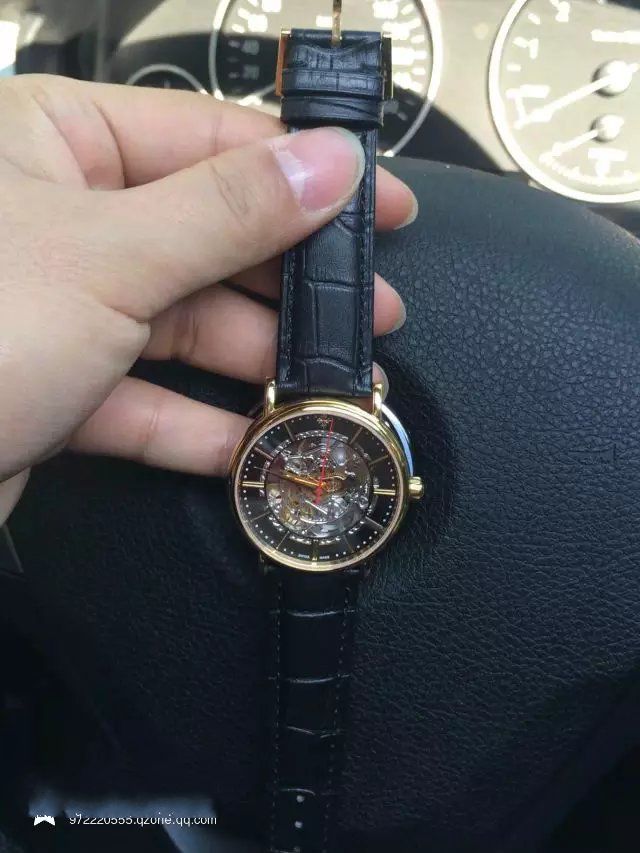In this detailed image, a person is showcasing a wristwatch while seated in a stationary car. The watch is held up against the steering wheel with their left hand, revealing their slightly long, natural nails. The timepiece features a sophisticated design with a black leather band and a black and gold face embellished with intricate lines and dots, eschewing traditional numbers. In the background, the car's speedometer and odometer are visible, indicating the vehicle is parked and not running. A blurred-out watermark in the lower left corner discreetly conceals a phone number.